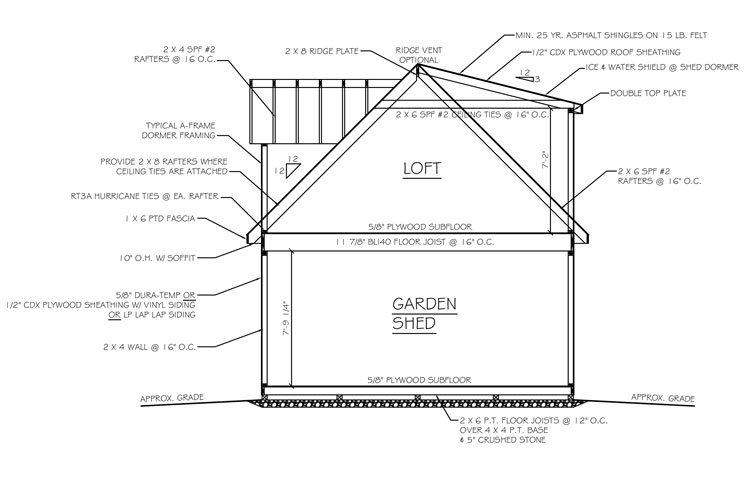Here is a refined and detailed caption for the architectural drawing:

---

This architectural drawing represents a detailed layout of a small building designed with multiple functional areas. At the base of the structure is a garden shed, while the upper section features a loft. An additional ridge plate is indicated for a secondary loft area. Each segment of the building is meticulously annotated with detailed specifications and measurements. The drafting specifies typical A-frame dormer framing using 2-by-6 number two-grade rafters. The roofing is designated to be covered with durable 25-year asphalt shingles. 

Measurements for the entire structure, including the beams, walls, and subfloor, are clearly delineated, providing precise dimensions and materials needed for construction. Plywood for the subfloor is also specified, ensuring a comprehensive guide for the building process. This detailed schematic encapsulates a thorough depiction of the building’s intended composition and structural elements.

---